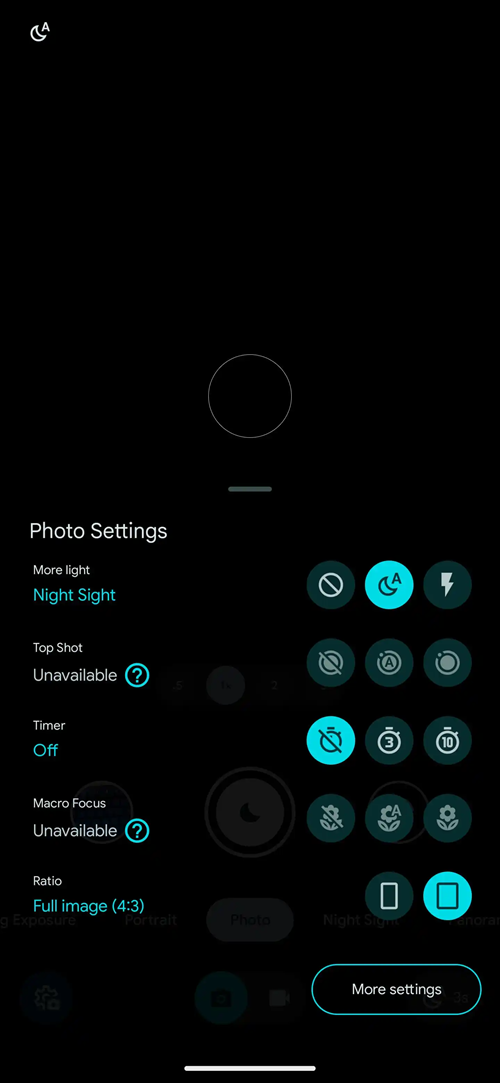The image depicts a camera app in dark mode, likely with the lens cover on, rendering the screen almost entirely dark. Centered on the screen is a circular crosshair graphic, suggesting that once settings are adjusted, the camera will be ready to operate. The photo settings menu displays several options:

- **Night Light Settings:** Can be toggled between Off, On, or Automatic mode, which uses a sensor to decide.
- **Top Shot:** Currently unavailable, indicated by a question mark which may suggest it requires an additional purchase or upgrade.
- **Timer:** Set to Off, but can be adjusted to 3 seconds or 10 seconds.
- **Photo Focus:** Unavailable in the current mode.
- **Image Ratio:** Set to Full Image for 3, referring to the aspect ratio of the photo.

The detailed settings imply a comprehensive and user-adjustable photo-capturing experience.